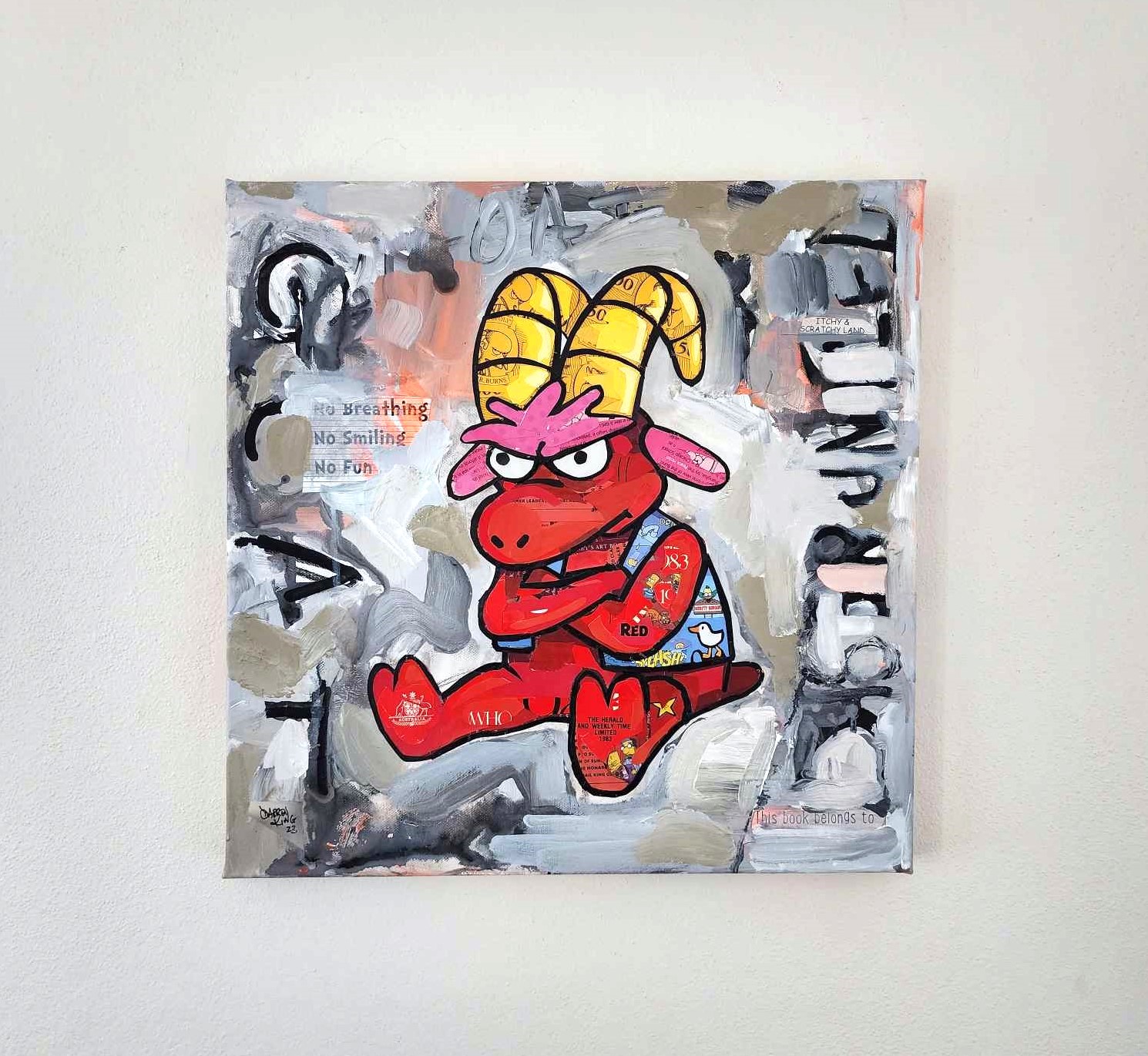The image is a vibrant, modern art depiction of a cartoon-like, red goat character with gold/yellow horns and pink ears and hair, set against a textured background of gray, beige, and pink hues, created using a mix of graffiti-like brushstrokes and potential finger-painted elements. The red goat, which exudes a grumpy demeanor with crossed arms, wears a blue denim vest adorned with various designs, including a duck. Notably, the painting incorporates a collage technique, featuring elements like the Simpsons characters on the goat's horns and text references such as "Itchy and Scratchy Land." Prominent textual elements within the artwork state, "No Breathing, No Smiling, No Fun" and "This Book Belongs To" — the latter left unnamed. Additionally, there is a faint, partially obscured inscription that appears to read "83" and a signature resembling "King 23." A bird is subtly integrated into the graffiti, enhancing the layered complexity of the piece. The overall presentation resembles a canvas composition hanging on a stark white wall, merging painting and collage art forms cohesively.